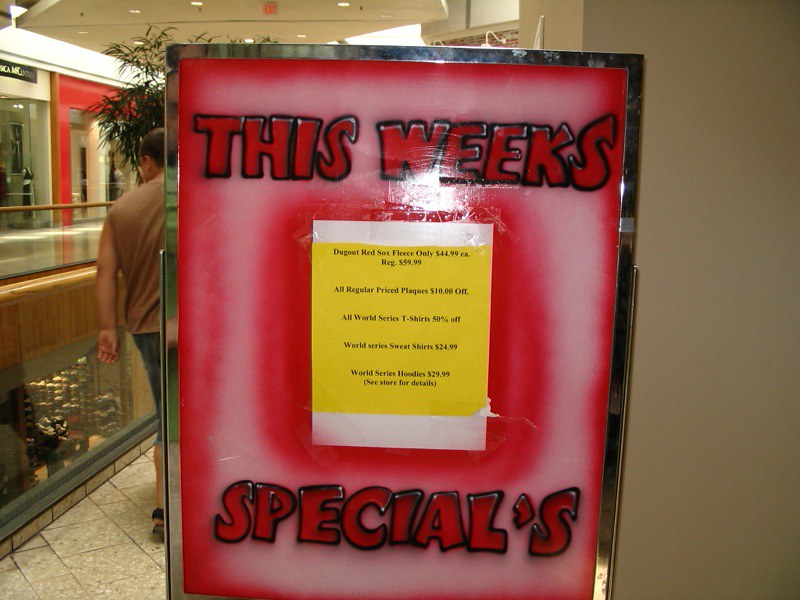This detailed caption describes a photograph of a bustling indoor mall, focusing particularly on a handmade sign. The sign, prominently displayed within the mall, is rectangular and bordered by a silver metal edge visible on the top, right, and left sides. The main text on the sign reads "This Week's Specials" in bold block letters, with "This Week's" positioned at the top and "Specials" at the bottom. The letters are strikingly red with a black outline, set against a backdrop of red and pink. Between these lines of text is a yellow paper insert, listing various sale items related to the Red Sox, a well-known baseball team.

In the upper right portion of the image, a reflection can be seen, adding a layer of dimension to the scene. To the left of the sign, a man stands out; he is dressed in a sleeveless brown t-shirt, long denim shorts, and sandals. He has short brown hair and appears to be gazing down. This indicates that the mall is multi-leveled, and the man seems to be observing a shoe store on the lower level. The image captures a moment of everyday activity within the shopping center, highlighting both the promotional sign and the casual interactions of shoppers.